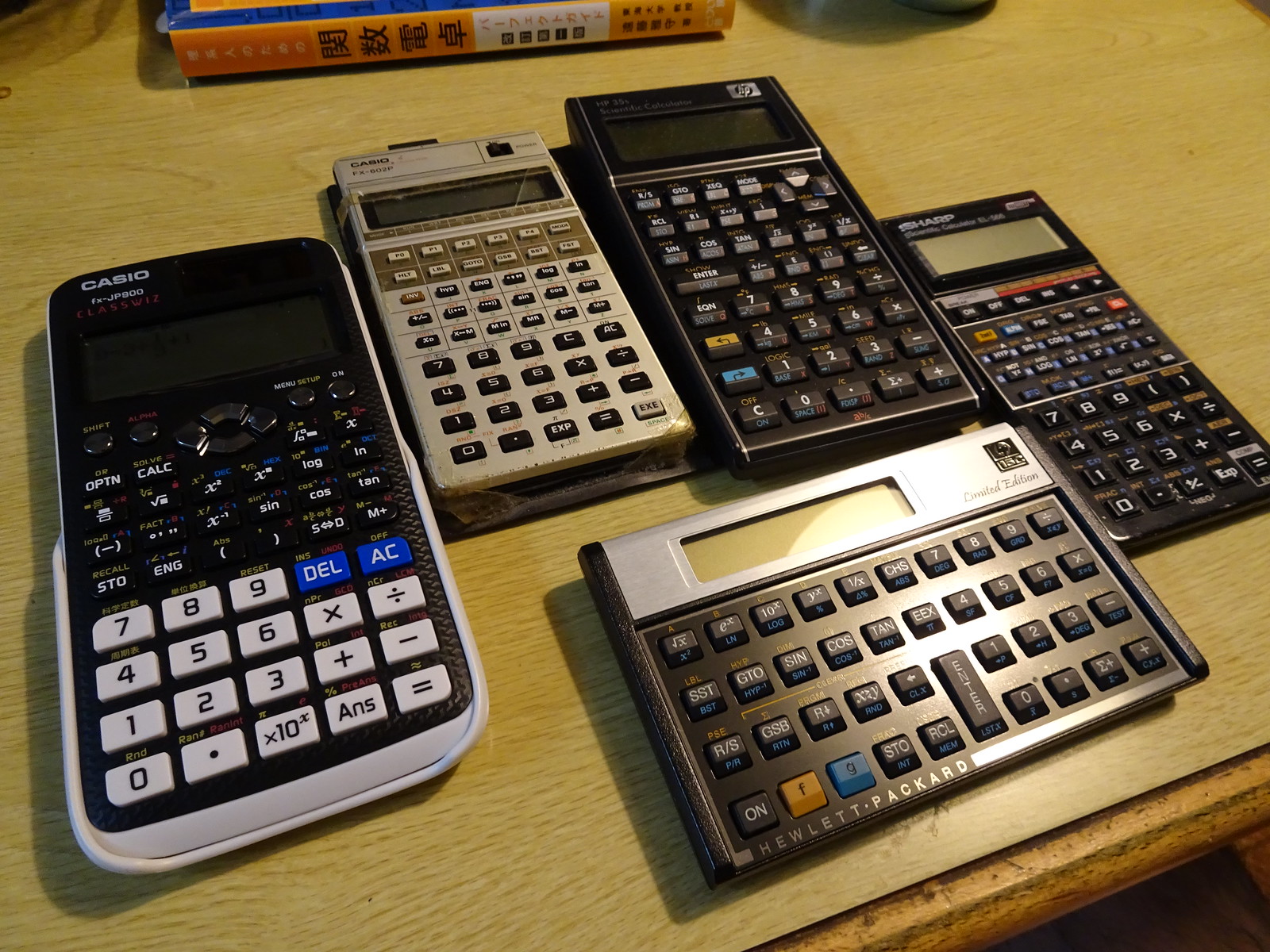The image depicts a collection of five calculators arranged on a light brown, school desk-type surface. At the top of the scene, two books with Chinese lettering are faintly visible. The calculators, primarily scientific in function, form a loose pattern. In the top left corner, two Casio calculators sit side by side, with their brand names more or less prominently displayed at the top. To their right is an HP-branded calculator, followed by a Sharp calculator positioned next to it. The fifth calculator, situated at the bottom, is horizontally aligned and bears an indistinct logo but is identifiable by the text "Hewlett Packard" at the bottom. While one of the calculators appears to be brand new, the remaining four show varying levels of use, with one looking particularly well-worn. Each calculator varies in color and button configuration, highlighting their diverse functionalities.